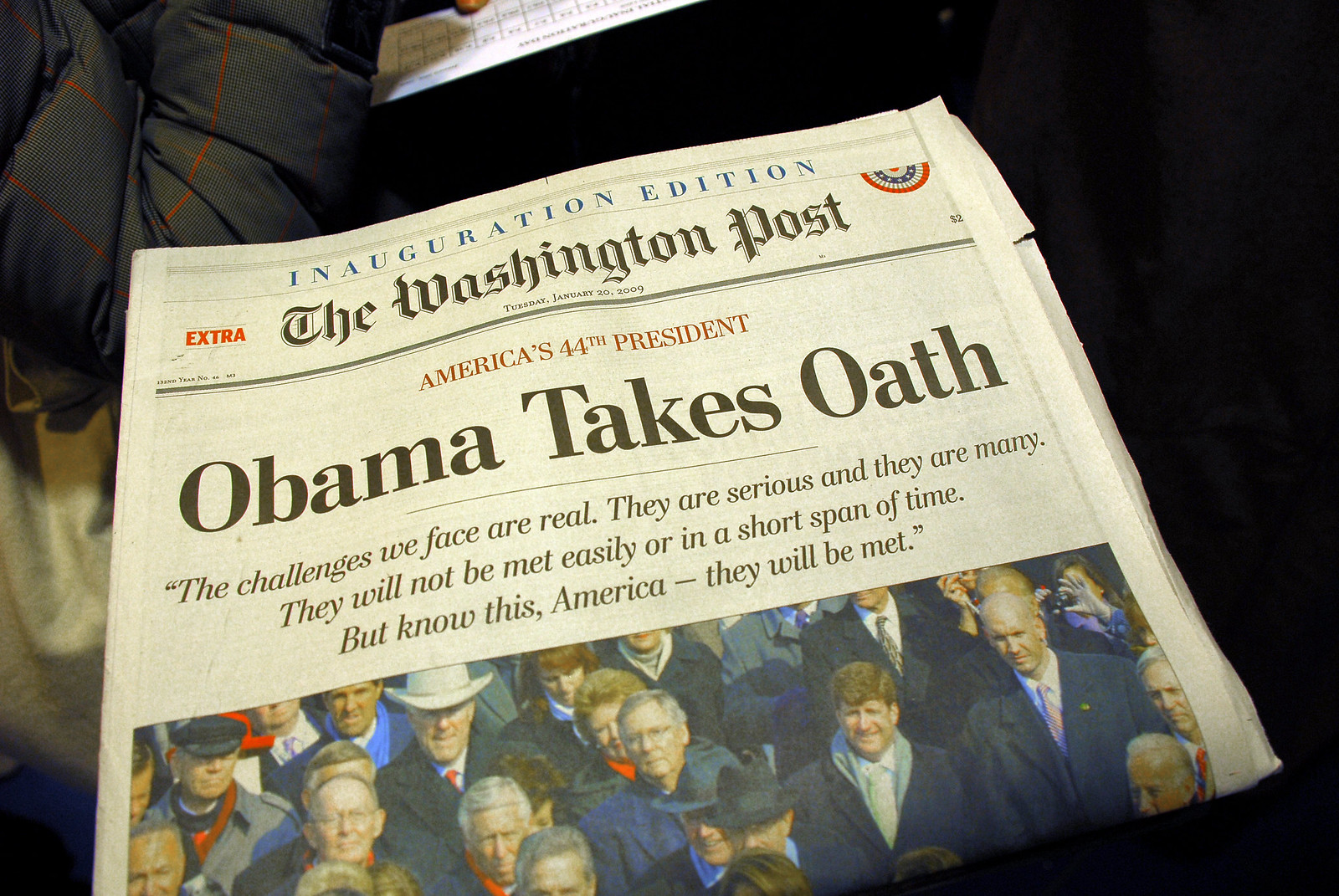The image depicts the front page of an Inauguration Edition of The Washington Post, with a dark background, likely black fabric or jacket, suggesting it's lying on a bed or couch. At the top, in blue text, it reads "Inauguration Edition," followed by "The Washington Post" in black. Below a black divider line, red text proclaims "America's 44th President." The main headline in bold black letters states, "Obama Takes Oath," followed by a quote: "The challenges we face are real. They are serious and they are many. They will not be met easily in a short span of time. But know this, America, they will be met." Beneath the text is a photo of President Obama's inauguration, showing people in dark coats and hats, presumably senators and other officials, seated in the stands, all facing the same direction. The newspaper has a light gray hue characteristic of typical newsprint.